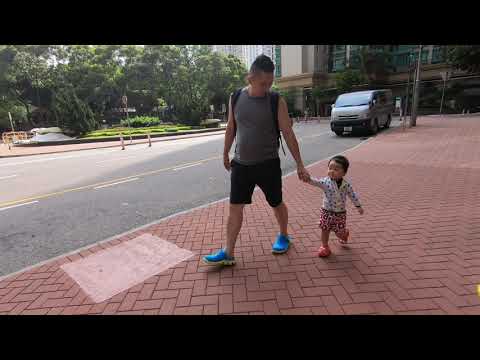A man wearing a gray sleeveless shirt, black shorts, and bright blue shoes, carries a backpack over his shoulders and has short black hair. He walks hand-in-hand with a toddler dressed in a white shirt with spots and red shorts with white designs. Similar to the man, the toddler wears sporty shoes, but in a pink or red color. They stroll together on a V-shaped interlocking brick sidewalk in a city, bordered by light red pavement. To their left, a roadway features a van parked a little ways behind them. Across the street is a lush green park with grass, bushes, trees, and some hedges, and the base of some buildings can be seen in the background.